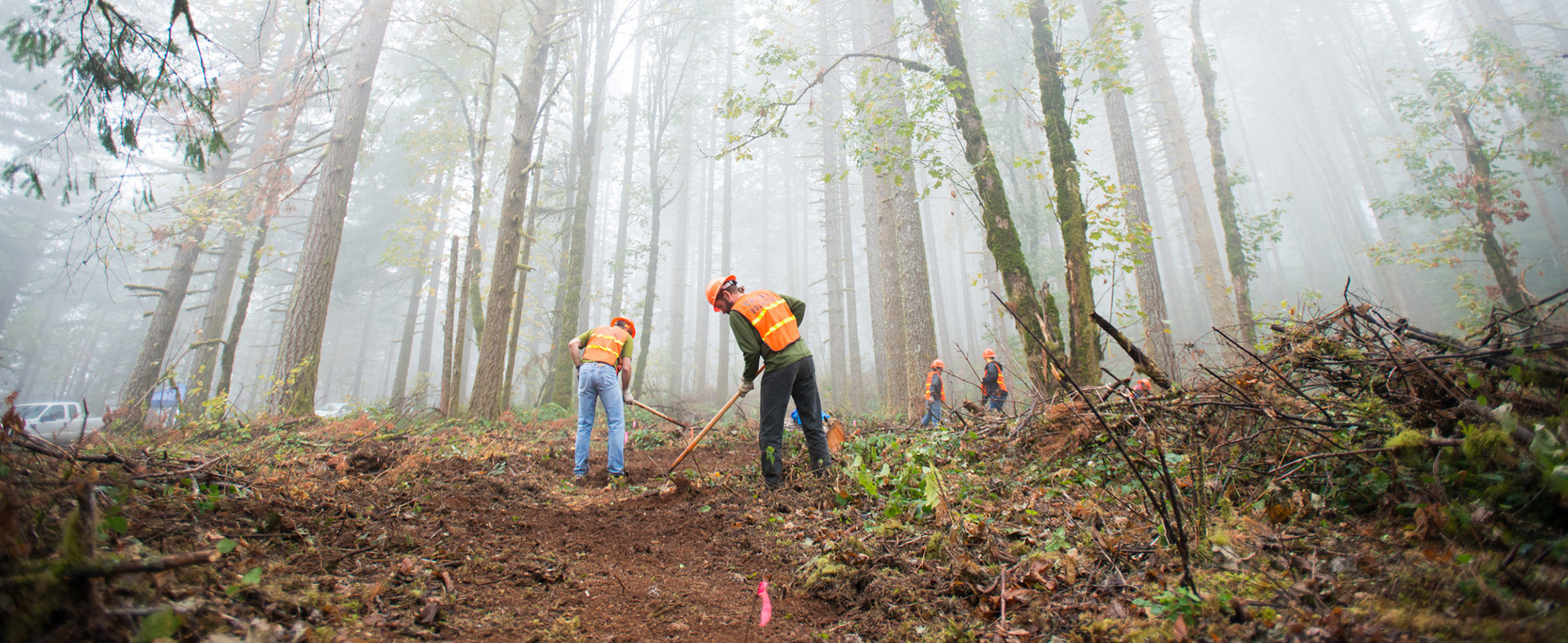In this detailed, outdoor photograph taken in a forest, the scene is shrouded in a light grayish haze or fog, giving it a misty atmosphere. The ground is mostly bare with hints of green vegetation, indicating it might be spring or summer. There are tall trees, showing only their lower trunks, adorned with green leaves. The focal point of the image is a group of men clad in orange safety vests with neon yellow stripes and matching orange hard hats. They are engaged in physical labor, using hoes and rakes, possibly to clear a pathway or create a firebreak. Some of the workers are visible in the background, similarly equipped and seemingly performing comparable tasks. Branches are piled up around the cleared ground, and small stakes with pink ribbons are scattered about, marking specific points. On the right side of the photograph, there is a white truck with another vehicle, maybe a white car, parked behind it. Further into the background, a large blue object is faintly visible between the trees, but its exact nature is unclear. This forest scene, almost devoid of grass, suggests an organized effort, possibly for forest maintenance or fire prevention.